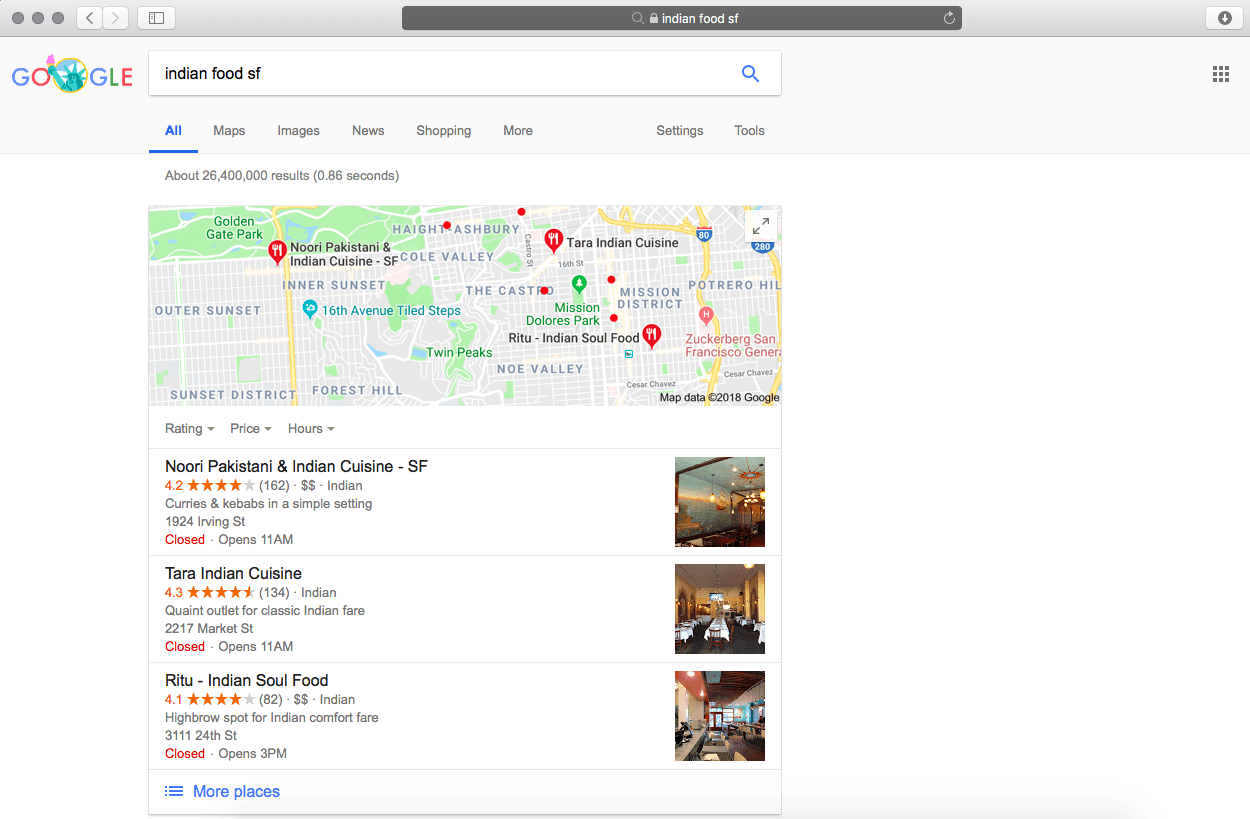This image depicts a Google search results page with a query for "Indian food SF." At the top of the screen, there's a dark gray navigation ribbon featuring a darker gray search bar with the query text "Indian food SF" in white. Below this, a lighter gray ribbon spans the width of the page, showcasing the word "Google" on the left—where the second "O" is replaced by an illustration of the Statue of Liberty. To the right of "Google," the search bar reiterates the query "Indian food SF" in white text.

Beneath this, the ribbon displays various search options: "All," "Maps," "Images," "News," "Shopping," and "More," with additional options "Settings" and "Tools" positioned on the far right. The "All" tab is selected, highlighted in blue and underlined.

Following the search options, the page presents a vertical list of restaurant search results accompanied by a map at the top. This map features red pins indicating the locations of the restaurants. The first restaurant listed is "Nori Pakistani and Indian Cuisine-SF," followed by "Tara Indian Cuisine," and "Ritu Indian Soul Food."